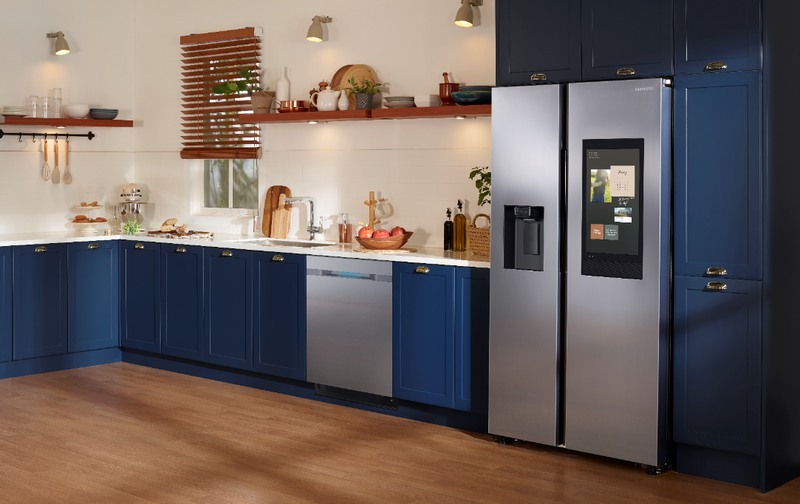This image features an indoor kitchen area with a streamlined and modern design. The floor is a warm wood type, possibly laminate, providing a cozy contrast to the dark navy blue cabinetry. The cabinets have elegant brass or gold pulls, adding a touch of sophisticated warmth, and are predominantly located on the lower part of the wall. Above the countertops, which are a pristine white, there is no cabinetry; instead, a single wooden shelf spans the length of the wall, adorned primarily with decorative items.

The kitchen includes a sleek, double-door refrigerator with a modern electronic touchscreen panel on one side, capable of handling notes, lists, and images. A wood blind covers the window above the sink, which is quite sizable and features a silver faucet. The lighting is embedded in the ceiling with canister lights ensuring the area is well-lit.

A silver dishwasher matches the refrigerator and sits neatly among the blue cabinetry. The appliance countertops are organized but busy, reflecting everyday use. Spoons hang from a bar on one of the shelves, adding a functional yet homey touch. There also appears to be a pantry cupboard adjacent to the fridge, ensuring ample storage space. The overall aesthetic is minimal yet functional, combining modern appliances with warm, earthy tones.